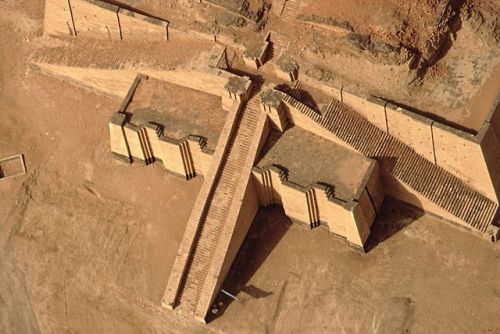The image showcases the base entrance of a ziggurat or pyramid, prominently featuring a straight flight of stairs leading up from a barren desert setting. The scene is dominated by hues of beige, brown, and yellow, characteristic of the sandy and dusty environment. The structure, composed of brownish-orange bricks and dirt, displays notable erosion at its top, though the lower sections and entrance stairs remain intact. There are three stairways ascending the structure, each separated by walls or barricades. Absent of windows, trees, or lettering, the image focuses on the stark, imposing nature of the staircase against the desolate background, suggesting an ancient, weather-worn edifice.